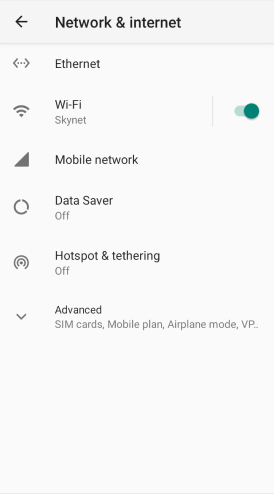This image is a screenshot from a smartphone displaying the "Network & Internet" settings menu. The interface has a clean, white background with black lettering, predominantly used for headings and icons.

At the top, there's a navigation bar with a left-pointing arrow, indicating a back button, and the title "Network & Internet" in bold black letters.

Directly below, there are various menu options for network-related settings:

1. **Ethernet**: Represented by an icon of dots connected with a line.
2. **Wi-Fi**: Displaying the text "Wi-Fi Skynet" alongside a Wi-Fi icon, indicating that Wi-Fi is currently enabled with a green toggle.
3. **Mobile Network**: Marked by a signal strength icon and the label "Mobile Network".
4. **Data Saver**: Indicated by a broken circle icon with the text "Data Saver Off".
5. **Hotspot & Tethering**: Signified by a hotspot icon with the status "Hotspot Tethering Off".

Towards the bottom of the menu, there's an expandable "Advanced" section, identified by a down arrow. Under this section, the options include:
- SIM Cards
- Mobile Plan
- Airplane Mode
- VPN

This comprehensive menu allows users to manage various aspects of their smartphone’s network and internet connections.